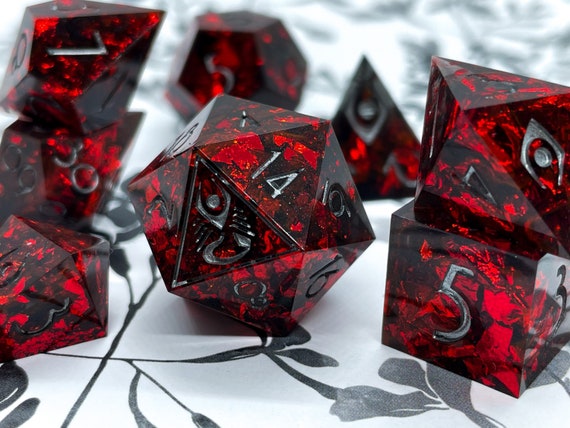This close-up photograph captures a collection of dice scattered across a white table adorned with black floral patterns. The dice are predominantly a dark red, marbled material, and are etched with silver numbers and symbols, including some resembling ancient Greek characters. The dice come in a variety of shapes, ranging from traditional cubes to more complex polyhedral forms, such as triangular and diamond configurations. Numbers visible on the dice include 1, 3, 5, 7, 14, 16, and 30, suggesting they are specialized pieces likely used in a board or role-playing game. The detailed shot emphasizes the intricate design and color contrasts of both the dice and the tablecloth.